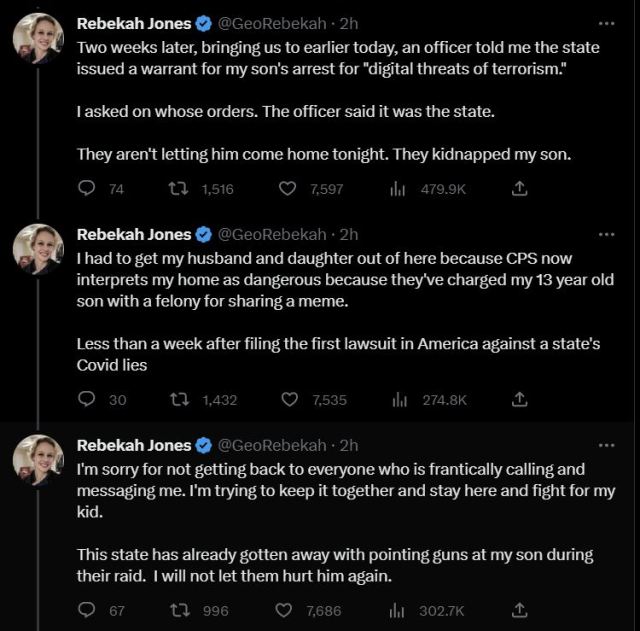In the image, the entire background is a solid black square. On the left side of the image, there is a circular profile picture of a female user named Rebecca Jones. Her name is displayed in blue text with a black check mark next to it, indicating verification. Her username is written as @GeoRebekah.

Rebecca Jones has made three consecutive posts:

1. "Two weeks later, bringing us to earlier today, an officer told me the state issued a warrant for my son's arrest for digital threats of terrorism. Based on whose orders? The officer said it was the state. They are letting him come home tonight. They kidnapped my son."

2. "I had to get my husband and daughter out of there because CPS now interprets my home as dangerous. This is because they charged my 13-year-old son with a felony for sharing a meme. Less than a week after filing the first lawsuit in America against a state's COVID lies."

3. "I'm sorry for not getting back to everyone who is frantically calling and messaging me. I am trying to keep it together and stay here and fight for my kid. The state has already gotten away with pointing guns at my son during the raid. I will not let them hurt him again."

These posts reflect a deeply personal and distressing situation involving state actions against her family.